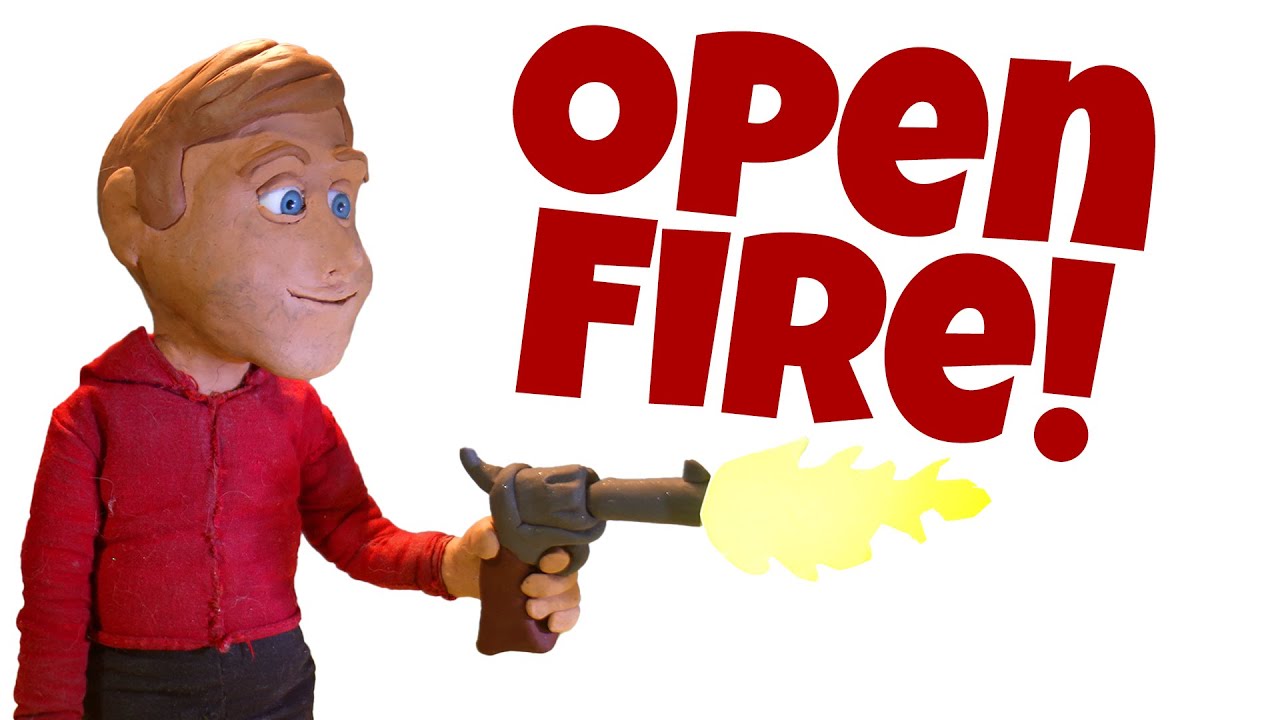The horizontal rectangular image appears to be an advertisement or a scene from a clay animation, featuring a clay figure of a young man or boy. Positioned on the left side, the clay figure has blue eyes and brownish hair, and is dressed in a red long-sleeved hoodie or jacket and dark pants. In his hand, he holds a clay revolver with a bright yellow and white flame coming out of the barrel, which appears to be digitally added. The dramatic action is heightened by large bold red letters on the right side of the white background that say "OPEN FIRE!" with an exclamation point. The entire scene captures the intensity and dynamism typically found in animated or cartoon advertisements.